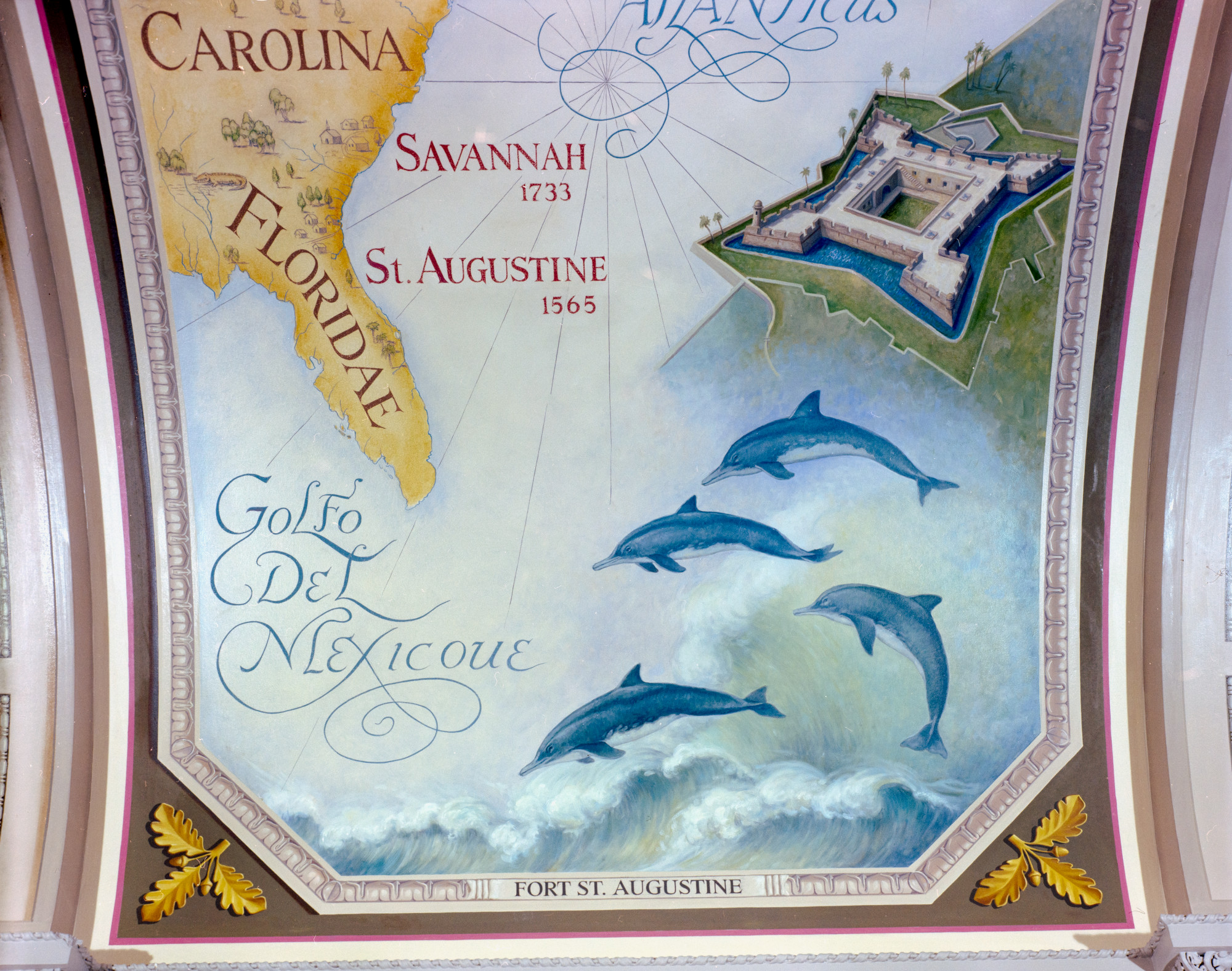This is a detailed color photograph depicting a framed, old-fashioned map of the southeastern coast of the United States, prominently featuring the Gulf of Mexico, labeled as "Golfo del Mexico." The core part of the image is a curved upper wall panel adorned with artistic details. Two white stone pillars frame the sides of the map. The map highlights several geographic and historical markers, including a yellow depiction of Florida, labeled "Floriday" and "F-L-O-R-I-D-A-E," with "Carolina" written above it. Additional labels include "Savannah, 1733," and "St. Augustine, 1565." An unusual, uniform-shaped building is illustrated at the upper right corner. At the bottom of the panel, four dolphins are drawn leaping above the water, adding a decorative touch to the scene. The bottom of the map also states "Fort St. Augustine" and is adorned with sprigs of yellow leaves on both the bottom left and right sides.